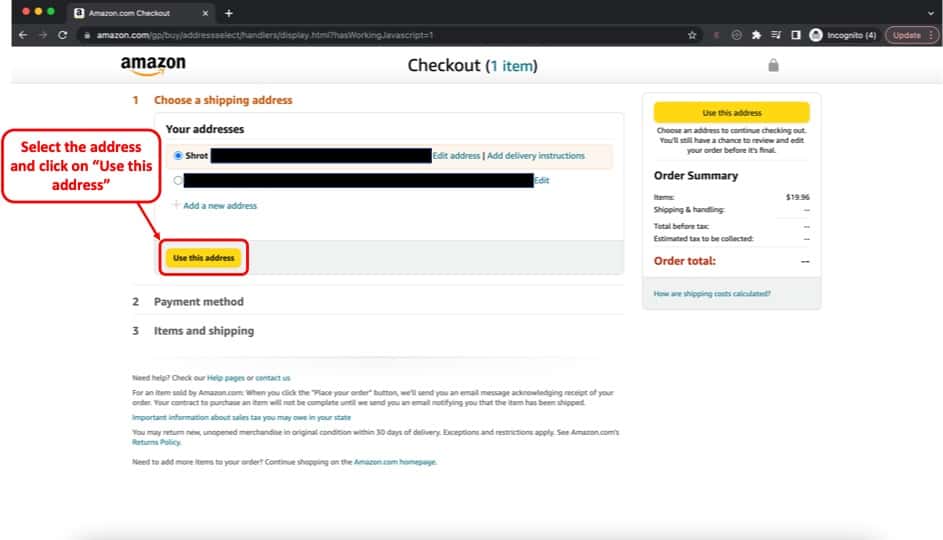This is a detailed screenshot of the Amazon.com checkout page, viewed through the Chrome web browser on a Mac. The browser window displays a single active tab showing the Amazon logo and the text "Amazon.com Checkout," indicating that the user is in the process of finalizing a purchase. There are also four incognito tabs open in the background.

The Amazon checkout page itself has a clean, white background, consistent with Amazon's typical website design. At the top of the page, the Amazon logo is prominently displayed, followed by the word "Checkout." Below this header, a blue-highlighted section indicates that the user is currently on the checkout page.

The page is organized in a step-by-step format. The first step, highlighted with an orange number "1," instructs the user to "Choose a shipping address." Below this heading, there is a section labeled "Your Addresses," where existing addresses have been blurred out for privacy. The user can select from two existing addresses or opt to "Add a new address."

To the right of these options is a prominent yellow button with black text that reads "Use this address." To ensure the user follows the correct procedure, there is a red-framed communication box to the left of this button. The box contains a red arrow and instructions in red text, directing the user to "Select the address and click on 'Use this address.'"

Once the user selects an address, they will proceed to additional steps such as choosing a payment method and confirming their items and shipping details.